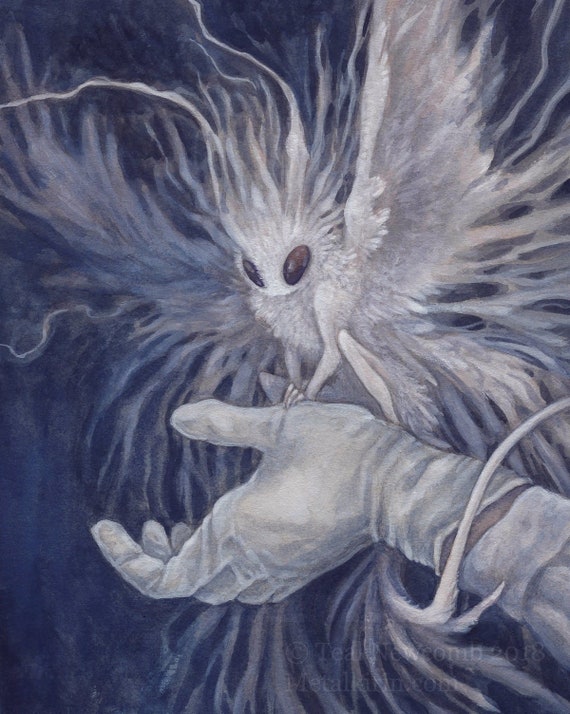The image depicts an artistic illustration of a strange creature perched on an outstretched, gloved hand emerging from the bottom right corner of the composition. The creature, reminiscent of a moth or fairy, possesses large oval-shaped eyes, primarily black but sometimes described as brown. Its insectoid face contrasts with its long, wispy wings and feather-like appendages. The white glove covers the thumb and first finger prominently, indicating the hand is positioned facing left. The artwork predominantly uses black, gray, and white tones, with some subtle hints of blue. The creature has a tail-like appendage wrapped around the wrist of the gloved hand. At the bottom of the image is a watermark stating "Teal New Comp 2018" and a barely legible URL, possibly "metalKirin.com."